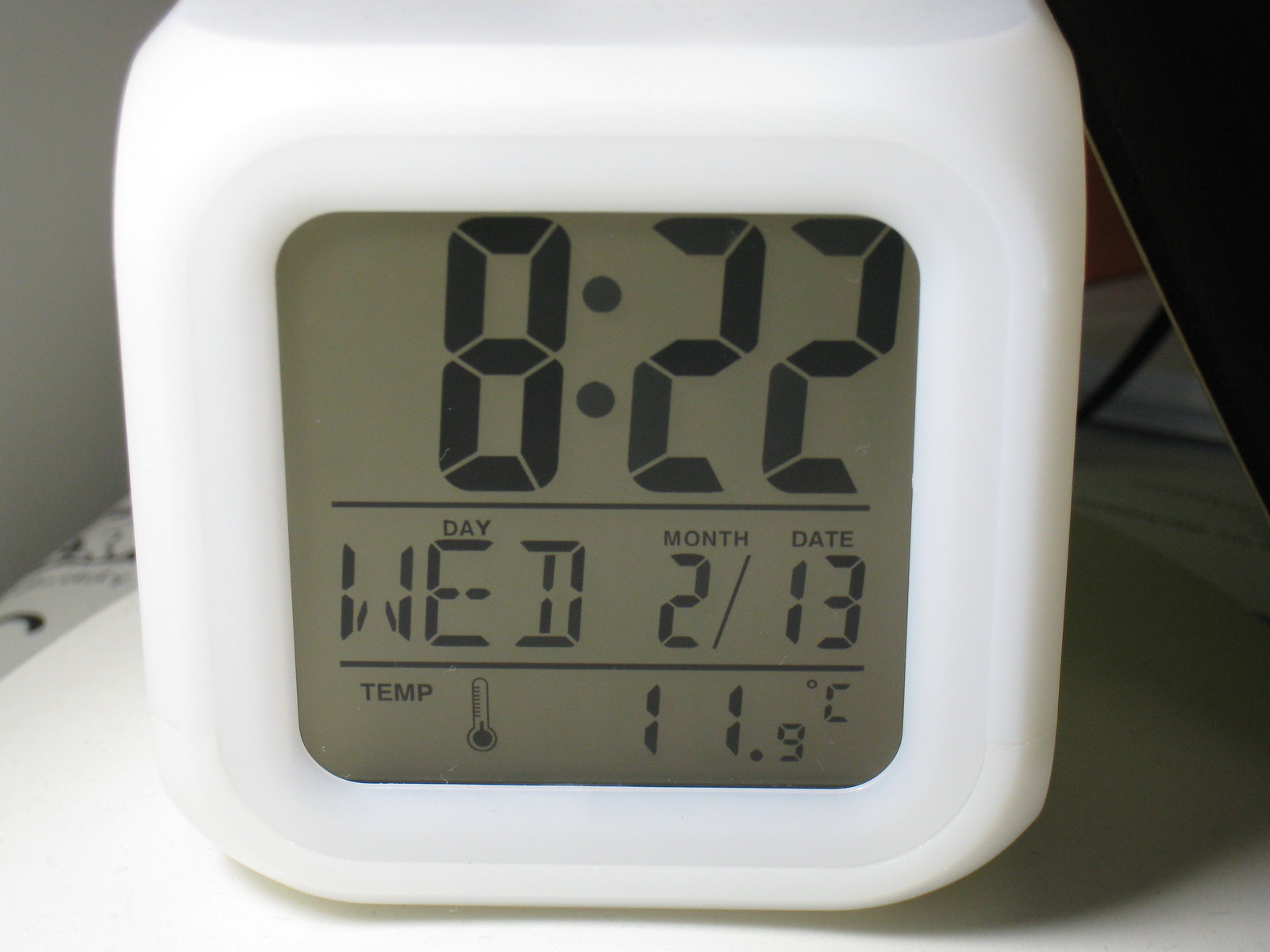A close-up image reveals a compact, white digital clock with a square design, bordered by a white plastic frame. The clock sits on a table, possibly resting on a piece of paper or a shell, with subtle shadows cast beneath it. The display features black numbers and letters on a gray screen. The largest numbers at the top indicate the time as 8:22, with a line underneath. The middle section shows the day and month with "Wed" for Wednesday, and the date "2/13" for February 13th. The bottom row displays the temperature, marked with a thermometer icon, reading 11.9°C.